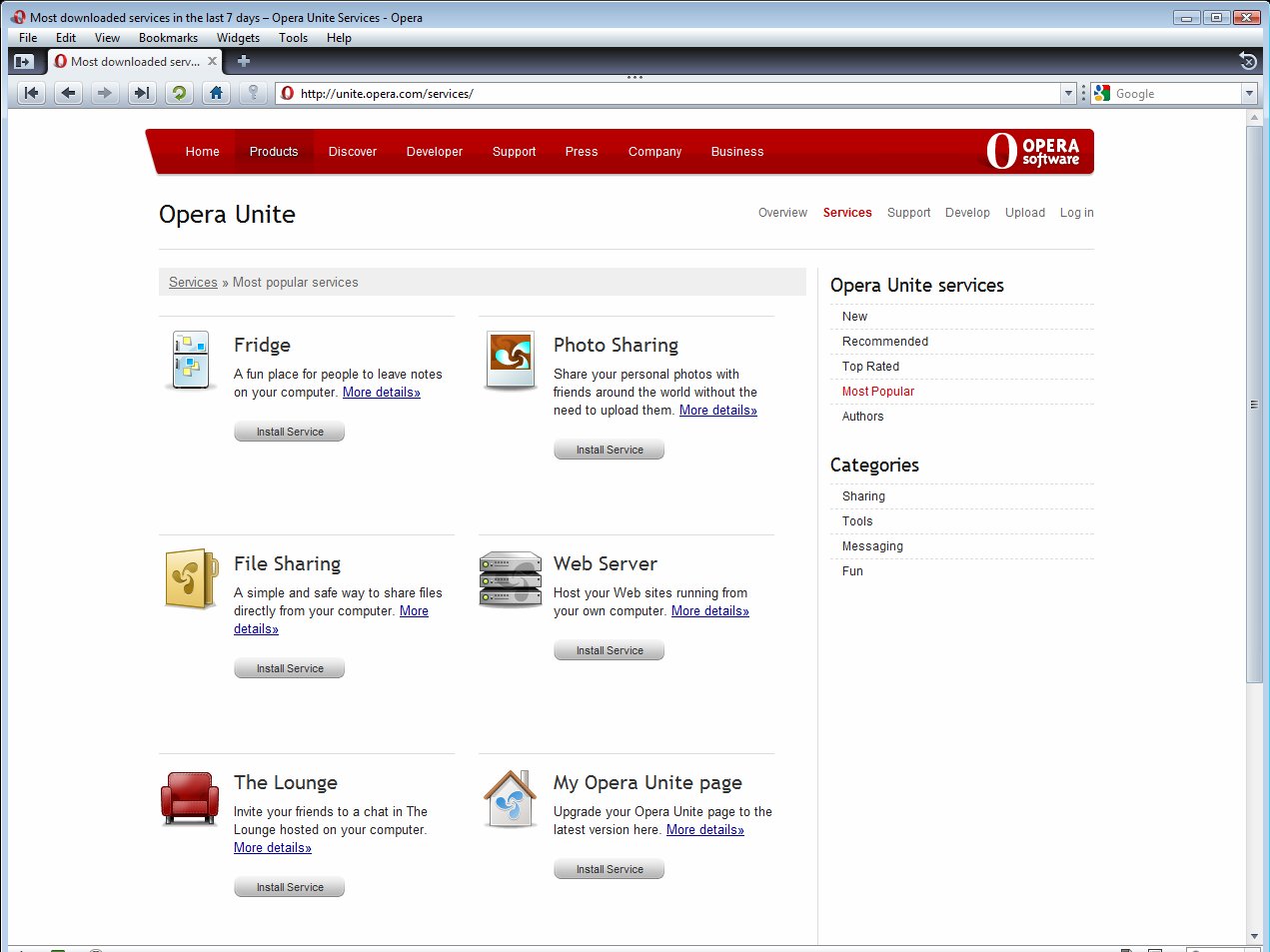This image is a screenshot of a website displayed on a desktop. The website features prominently the logo of Opera Software, with a red heading bar that spans the top of the page. The webpage is centrally justified on a plain white background, using a simple Arial font which makes the content straightforward and easy to read. The only splashes of color on the page come from the red heading bar and a series of small, colorful icons.

Six distinct icons are showcased below the heading bar, each representing different functionalities of the website. These icons include:

1. **Fridge**: This icon leads to a section described as a fun place for people to leave notes on your computer. A link is available for more detailed information.
2. **Photo Sharing**: This section allows users to share personal photos with friends globally, without the need for uploading them to a separate server. More details are accessible via an additional link.
3. **File Sharing**: It offers a simple and secure method to share files directly from the user's computer.
4. **Web Server**: Represented by another icon, although no additional descriptive text is provided in the initial voice caption.
5. **The Lounge**: Just like the Web Server, the Lounge’s specific details are not provided in the voice caption.
6. **My Opera Unite Page**: Completing the set of icons, this section presumably offers personalized settings or information related to the user's Opera Unite experience.

Overall, the webpage's design is minimalist, with content and functionality clearly presented to the user, providing easy navigation through the different services Opera Software offers.